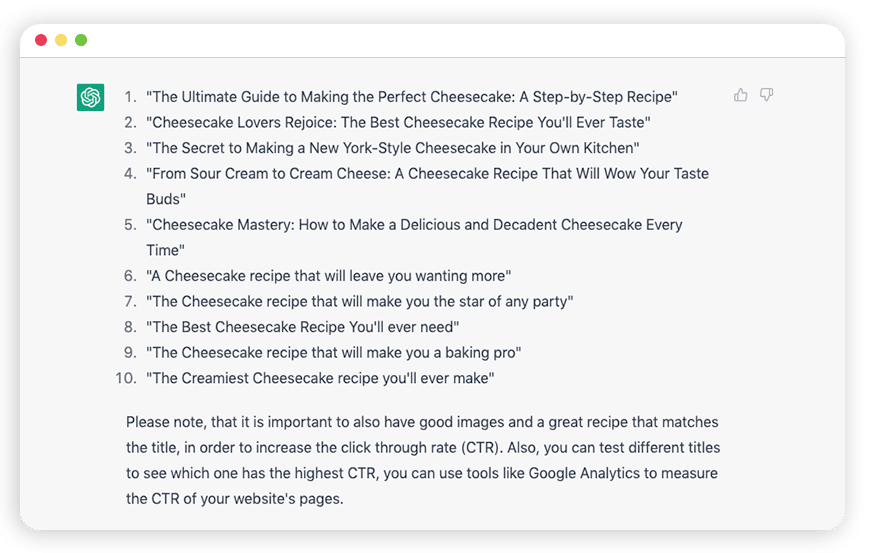The image features a minimalist design with three colored dots positioned in the upper left-hand corner: a red dot at the top, followed by a yellow dot, and a green dot at the bottom. Directly below these dots, there is a green square that contains a white icon resembling the top view of a flower.

Beneath the green square, a list of ten items is displayed, although only the first four and the odd-numbered ones from that point on are fully visible:

1. **The Ultimate Guide to Making the Perfect Cheesecake: A Step-by-Step Recipe**
2. **Cheesecake Lovers Rejoice: The Best Cheesecake Recipe You'll Ever Taste**
3. **The Secret to Making a New York Style Cheesecake in Your Own Kitchen**
4. **From Sour Cream to Cream Cheese: A Cheesecake Recipe That Will Wow Your Taste Buds**
5. **[Text not fully visible]**
...
8. **[Text not fully visible]**
10. **[Text not fully visible]**

A paragraph situated below the list advises that having high-quality images and a recipe that accurately matches the title is crucial for increasing the click-through rate.

The overall aesthetic is clean and organized, drawing the viewer’s attention to the sequence of articles on cheesecake recipes and tips for enhancing their attractiveness online.